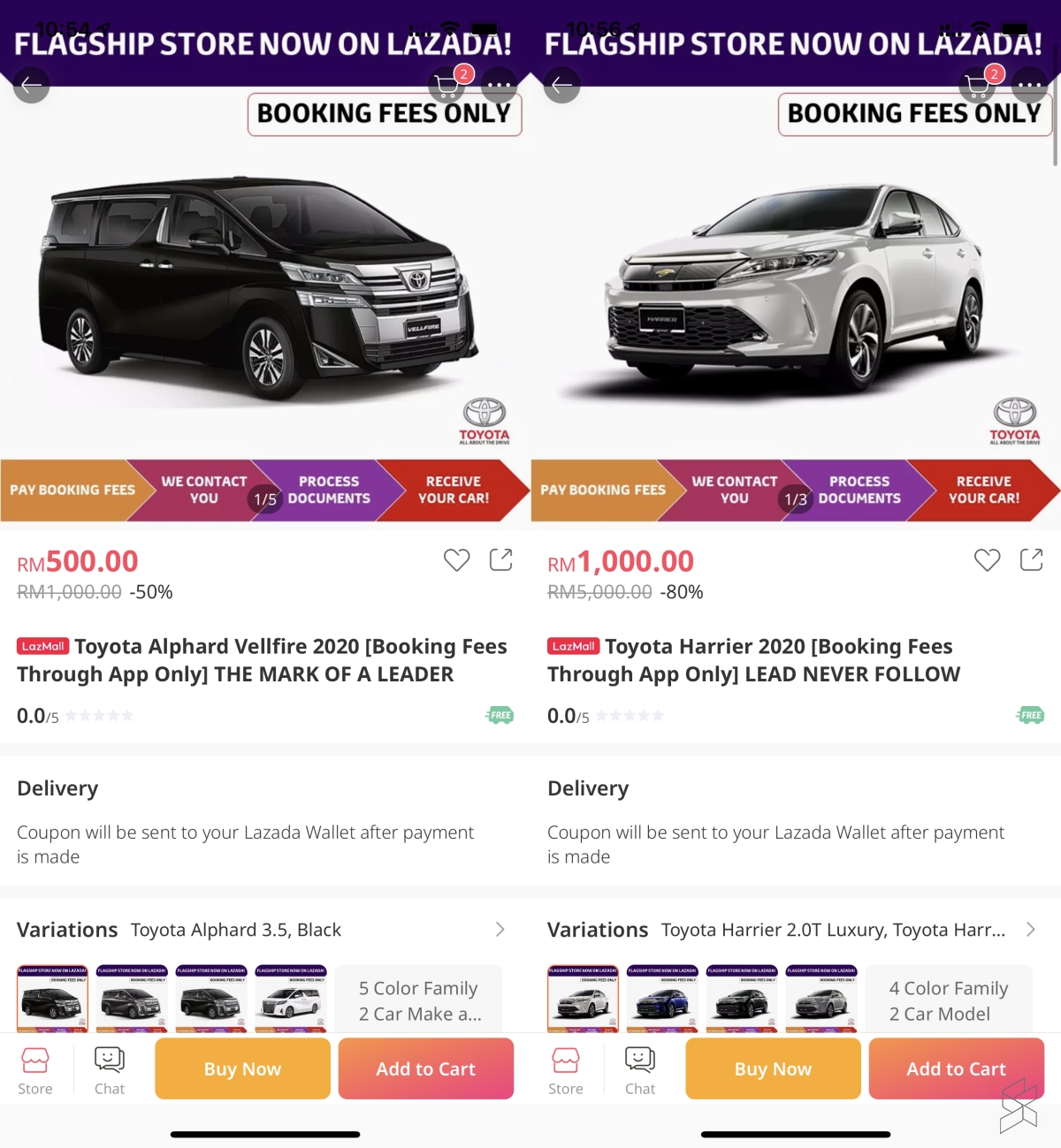**Detailed Caption:**

The image displays the user interface of a car rental store's web page, with two identical phone screenshots side by side. Each screenshot showcases the listings of two different cars available for rent.

At the top of both screenshots, there is a banner reading, "Flagship Store now in LASDA" highlighted in purple. Beneath the banner, the text "Booking Fees" is prominently featured in black. Each listing details a specific routine for the car rental process through clear menu options: "Pay Booking Fees," "We Contact You," "Process Documents," and "Receive Your Car." Each step is color-coded- the first step is highlighted in yellow, while the subsequent steps are in burgundy, purple, and red with white lettering.

On the left screenshot, a large image of a Toyota Alphard Vellfire 2020 model is displayed. The rental price is shown as RM 500, marked down from the original price of RM 1,000, reflecting a 50% discount. Additional information indicates that the booking fees apply for app users only, and a review rating is noted as 0.05 out of 5 stars. Upon payment, a delivery coupon will be sent to the LASDA wall. The model variations available are the Toyota Alphard 3.5 in black. Call-to-action buttons, "Buy Now" in yellow with white text, and "Add to Cart" in a red bar with white text, are present. There are also options for "Store" and "Chat" on the left side of the interface.

The right screenshot features the Toyota Harrier 2020 model, listed at a rental price of RM 1,000. This listing also follows the same structured layout with similar delivery and variation options, specifically the Toyota Harrier 2LT Luxury variant. The call-to-action and additional interface options remain consistent with the previous listing.

This page is evidently tailored for users wanting to book rental cars, providing detailed information and user-friendly navigation options to facilitate the car rental process.